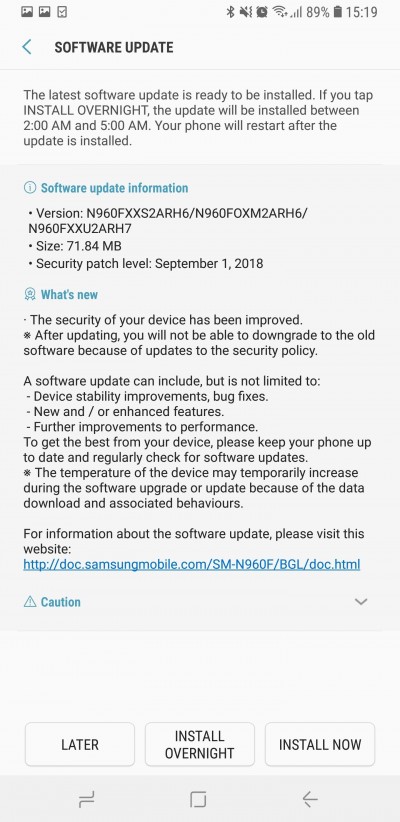The image depicts a smartphone screen displaying a software update notification. At the top, there are selectable images accompanied by a checkbox. Below this, typical phone status icons are visible, including Bluetooth, Wi-Fi, and battery indicators.

The second section features a blue back arrow alongside the text "SOFTWARE UPDATE" in uppercase letters. A message follows, stating, "The latest software update is ready to be installed." The phrase "INSTALL OVERNIGHT" is prominently highlighted in capital letters, informing the user that selecting this option will install the update between 2 a.m. and 5 a.m., with the phone restarting afterward.

Additional options are presented in blue text: "Software update information," "What's new," a clickable web link, and a caution icon with the word "caution" beside it.

Towards the bottom, there are three actionable buttons: "Later," "Install overnight," and "Install now." The very bottom row features the standard set of telephone icons.